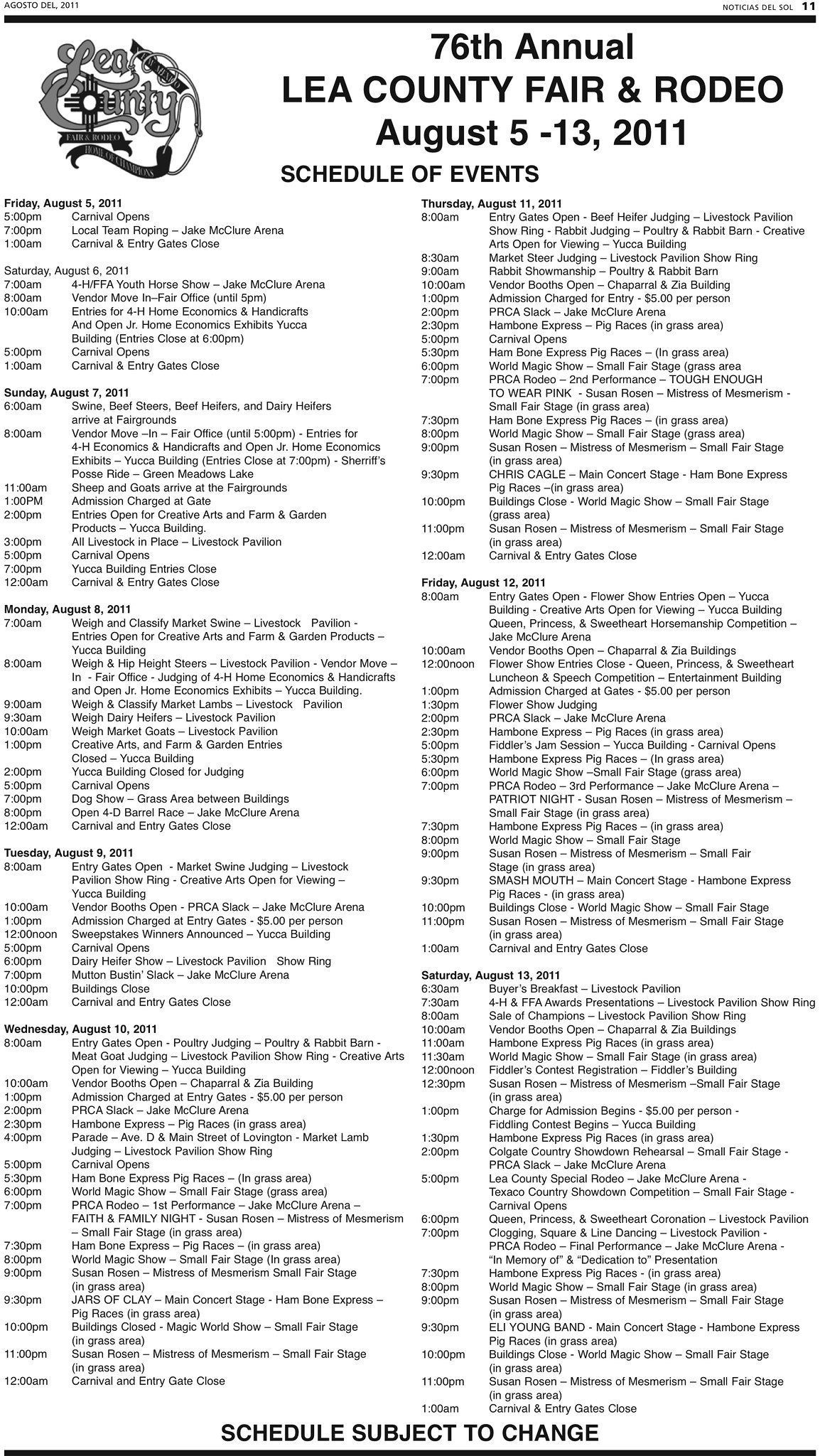The image features a detailed, black-and-white schedule of events for the 76th Annual Lee County Fair and Rodeo, held from August 5th through 13th, 2011. In the top left-hand corner, there is a decorative black and white cursive logo of "Lee County," designed with elaborate tails and wraparounds resembling vines. Adjacent to this, in bold text, it reads "76th Annual Lee County Fair and Rodeo." Directly below, in smaller font and centered, it states "Schedule of Events." The schedule is meticulously organized into two columns; the left column lists events from Friday, August 5th to Wednesday, August 10th, and the right column covers Thursday, August 11th to Saturday, August 13th. The text is very small, making it difficult to read specifics, but each day’s activities are itemized hour by hour. At the very bottom of the page, prominently displayed, is the notice "Schedule Subject to Change."